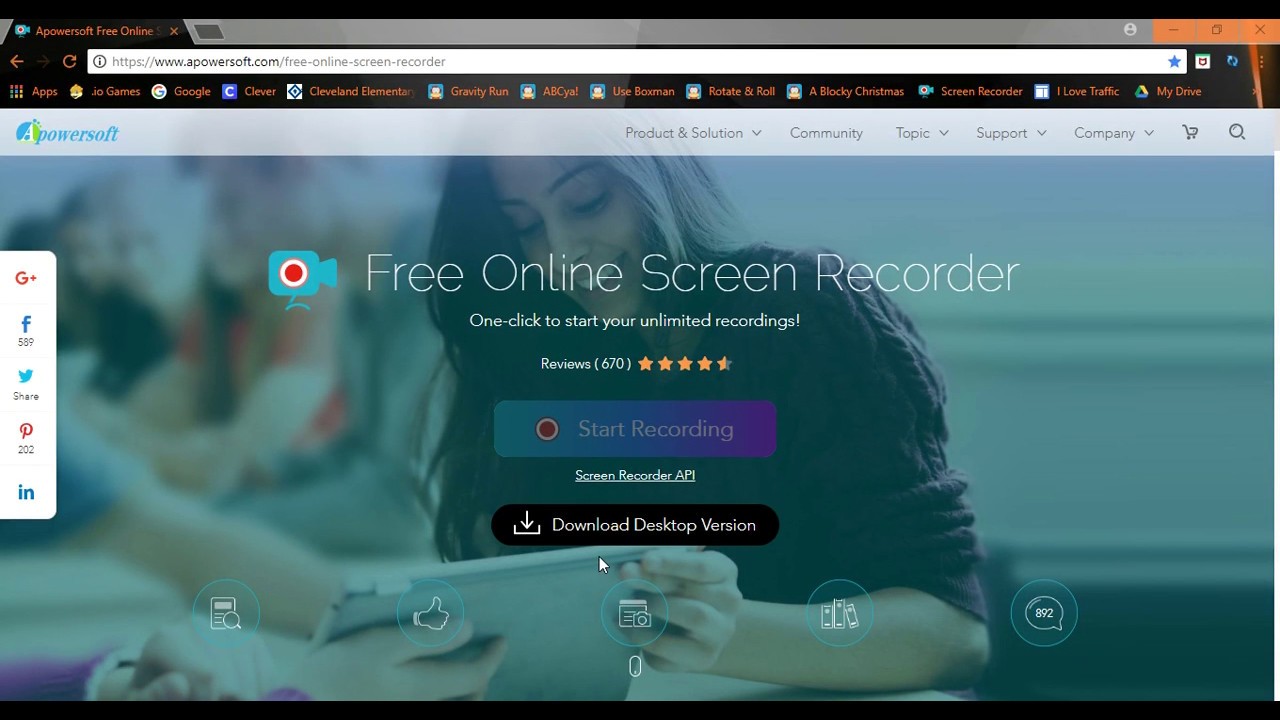This image features a detailed advertisement for PowerSoft's free online screen recorder, prominently displayed on a web page. The ad proudly boasts a user-friendly interface with a "One Click to Start Your Unlimited Recordings" slogan and an impressive user rating of four and a half stars from 670 reviews. 

In the background, a blurred, bluish-tinted image depicts a woman and a man, both engaged with a tablet, ostensibly demonstrating the screen recording functionality. The woman, with long dark hair, is wearing a sweater with sleeves rolled up, while the man beside her sports a short-sleeved blue shirt. A third person, visible only by their forearms, is also supporting the tablet and dressed in a purple sweater.

At the top of the web page, the search bar contains the text “apowersoft.com free online screen recorder,” clearly identifying the product. Various navigation options such as "Product and Solution," "Community," "Topic," "Support," and "Company" are available for user exploration. The bottom section of the ad includes several icons, including a search icon, a thumbs-up icon, another search icon, an icon depicting three phones together, and the number 872, which might signify further interactive elements or additional reviews.